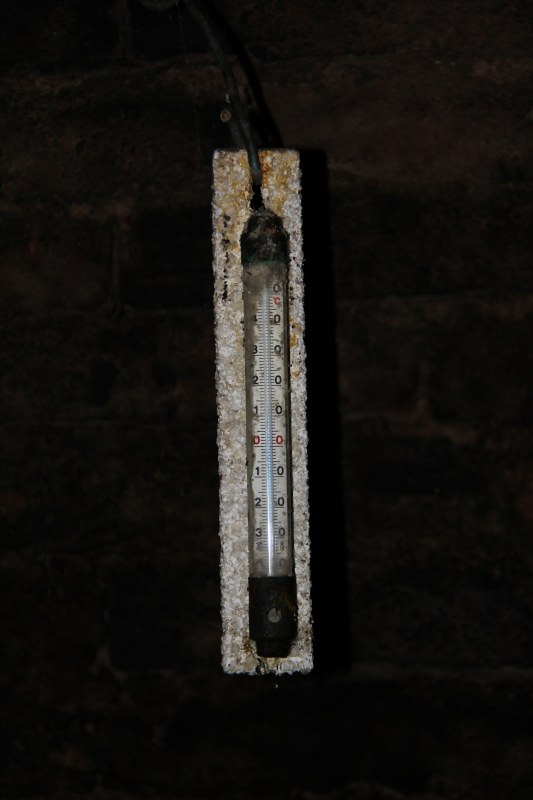This image depicts a neglected outdoor thermometer encased in what appears to be a white foam block. The thermometer is quite wide, with a clear body and black segments at both its top and bottom. It features a central zero marker, above which the inscribed numbers ascend—one, two, three—but these are only noticeable below the zero marker. The right side of the thermometer is obscured, with discoloration and dirt evident, suggesting a long period of disuse and outdoor exposure. The mounting mechanism, possibly plastic, is now ambiguous and heavily weathered, hinting at once-visible markings that have since worn away. The thermometer also shows signs of incompleteness, with the mercury column seemingly missing, rendering it non-functional. The background is featureless, providing no additional context or color to the scene. Overall, the image conveys a sense of abandonment and the passage of time.